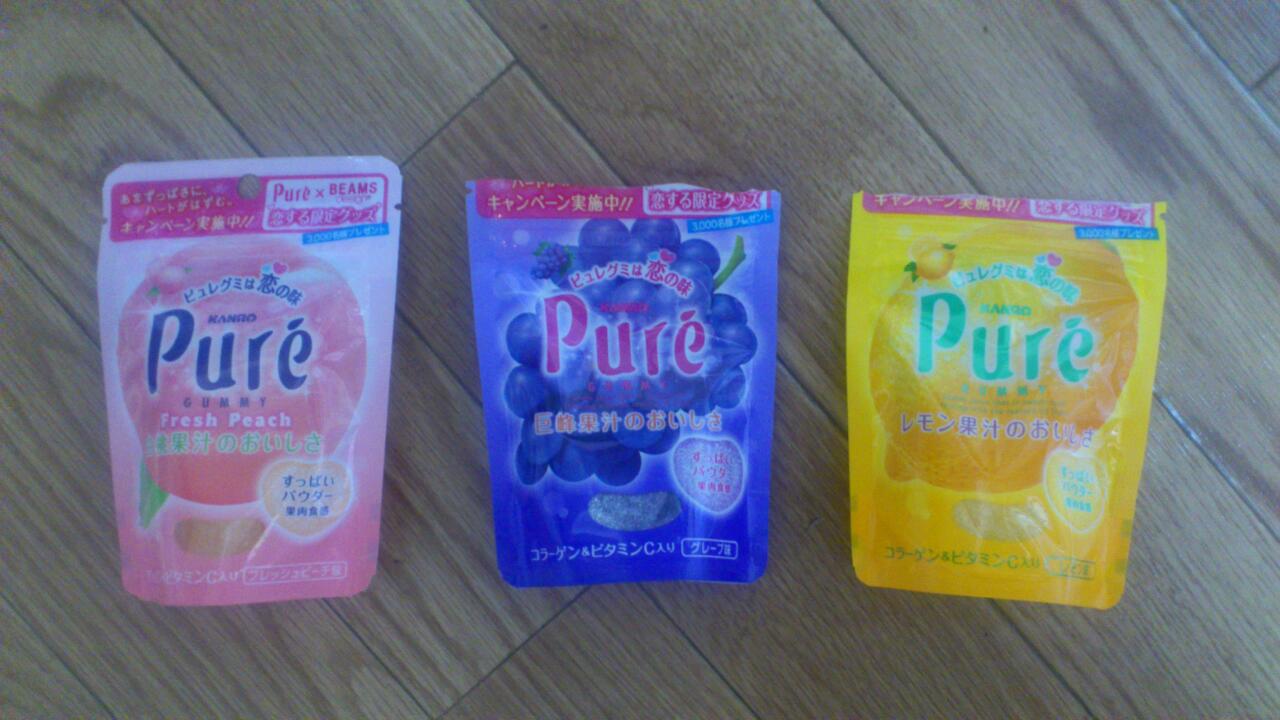This is an overhead color photograph of three Japanese gummy sweet packets, neatly lined up in a row with a small gap between each, on a wooden laminate floor displaying subtle bluish-grey tones. The packets, uniform in shape, feature the brand name "Pureé" with an accent over the 'e', along with Japanese script. The sweet flavors are fresh peach, purple grape, and lemon, each reflected in the packet colors: a pinkish peach on the left, a purple grape in the middle, and a yellow lemon on the right. The fruits are depicted on their respective packets—the peach packet showcases a large peach, the grape packet has a bunch of grapes, and the lemon packet displays a lemon. Notably, the pink peach packet appears unopened, while the grape and lemon packets have their tops torn off, indicating they have been opened. The arrangement and content capture a vibrant array of colors and textures set against the wooden backdrop.